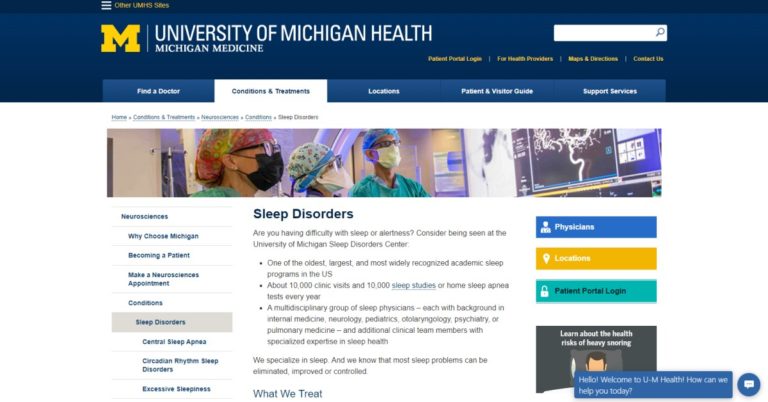The image depicts a detailed screenshot from the University of Michigan Health, specifically highlighting Michigan Medicine. The prominent yellow 'M' logo is visible, alongside text that reads "University of Michigan Health, Michigan Medicine." Below this header, menu options include "Find a Doctor," "Conditions and Treatments" (highlighted in white), "Locations," "Patient and Vendor Guide," and "Support Services."

The image prominently features a photo of three individuals wearing surgical masks and hair coverings, intently looking at a screen. To the left side of the image, there are sections titled "Neurosciences," with sub-options such as "Why Choose Michigan," "Become a Patient," "Make a Neurosciences Appointment," and a list of conditions, including "Sleep Disorders," "Central Sleep Apnea," "Cardiovascular Rhythm Sleep Disorders," and "Excessive Sleepiness."

On the right side, there is a focus on "Sleep Disorders" with text that reads: "Are You Having Difficulty With Sleep or Alertness? Consider Being Seen at University of Michigan Sleep Disorder Center." This is followed by a detailed description of the center, highlighting that it is one of the oldest, largest, and most widely recognized academic sleep programs in the U.S., with about 10,000 clinic visits and 110,000 sleep studies or home studies conducted annually. The center is staffed by a multidisciplinary team of sleep physicians with backgrounds in internal medicine, neurology, pediatrics, psychiatry, or pulmonary medicine, along with additional clinical team members who have specialized expertise in sleep health. The text emphasizes, "This is what we treat."